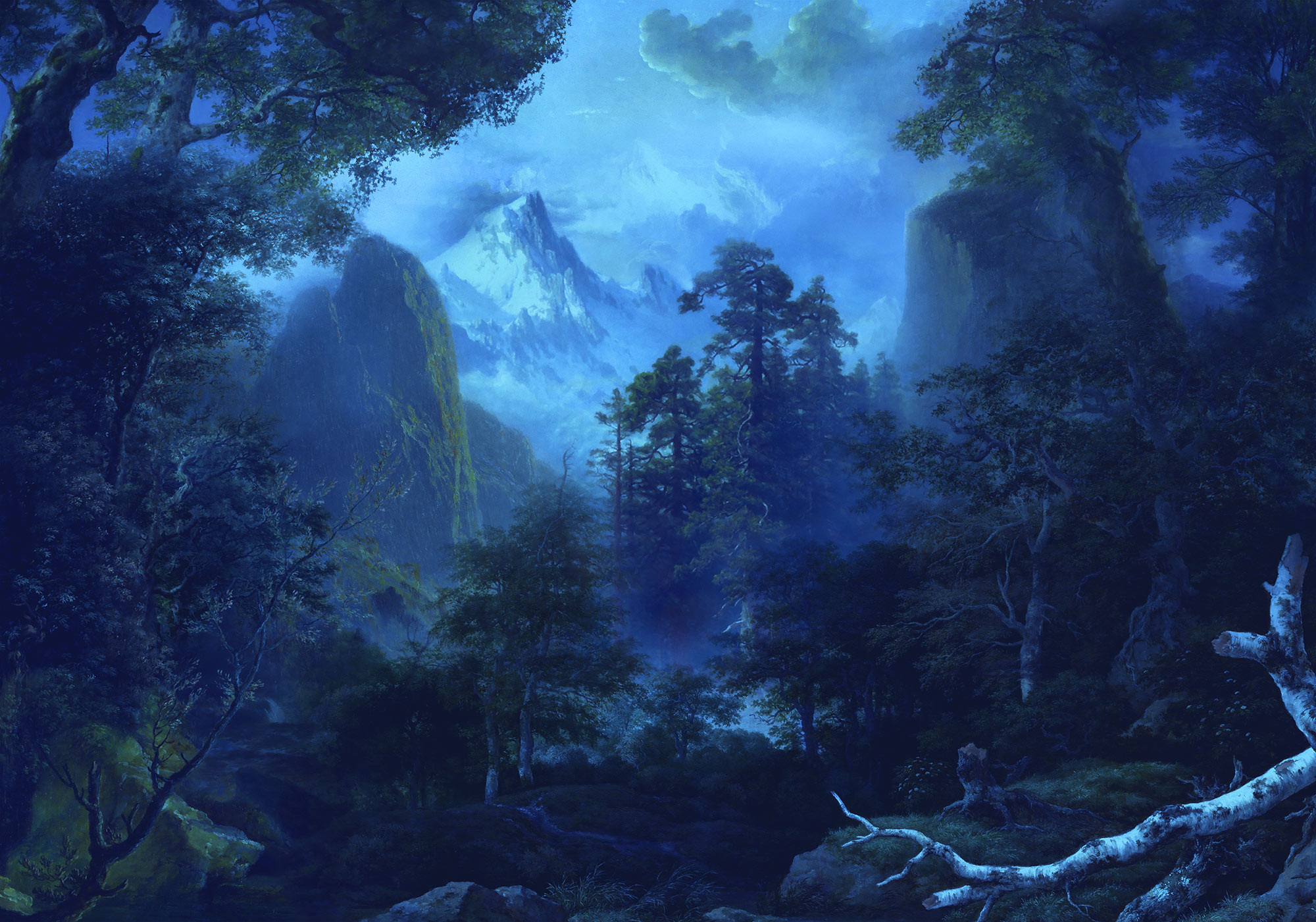The image portrays a dark, moody forest scene with a variety of natural elements layered throughout. In the foreground, a large fallen birch tree branch lies on the right side among numerous trees growing at various angles, suggesting a rocky terrain with rocks appearing to slope downwards. To the left, a towering dark boulder covered in green moss is prominent. Moving further into the scene, a patch of trees leads the eye towards a distant valley enclosed in fog. The background reveals mountains illuminated against the gloomy sky, seemingly snow-dusted with puffy white clouds above. The muted colors transition from blacks and dark greens to grays and blues, adding to the image's mysterious and almost painting-like quality.